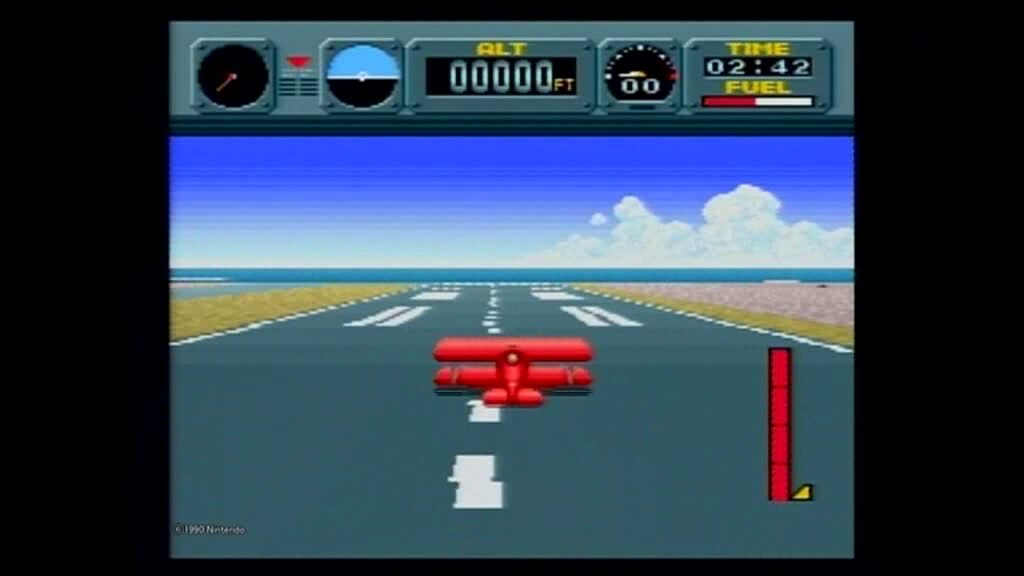This image is a screenshot of an older-style video game, specifically a flying simulator featuring a red old-fashioned biplane sitting on a gray runway with white lane stripes. The runway leads directly into a body of water, framed by green grass on either side. The sky above is blue with a few clouds, suggesting a clear day. At the top of the screen, detailed instrumentation is displayed: an altimeter reading 0000 feet, a fuel gauge at half capacity, and a time clock reading 2:42. Additionally, there is a life screen on the right side, colored red and showing four "R"s, indicating the remaining lives or attempts. Various other gauges, including one that seems to ensure the plane's level alignment, are cluttered in the upper left corner of the screen. The graphical style appears low-tech by today's standards, likely suggesting a nostalgic or retro aesthetic for the game.